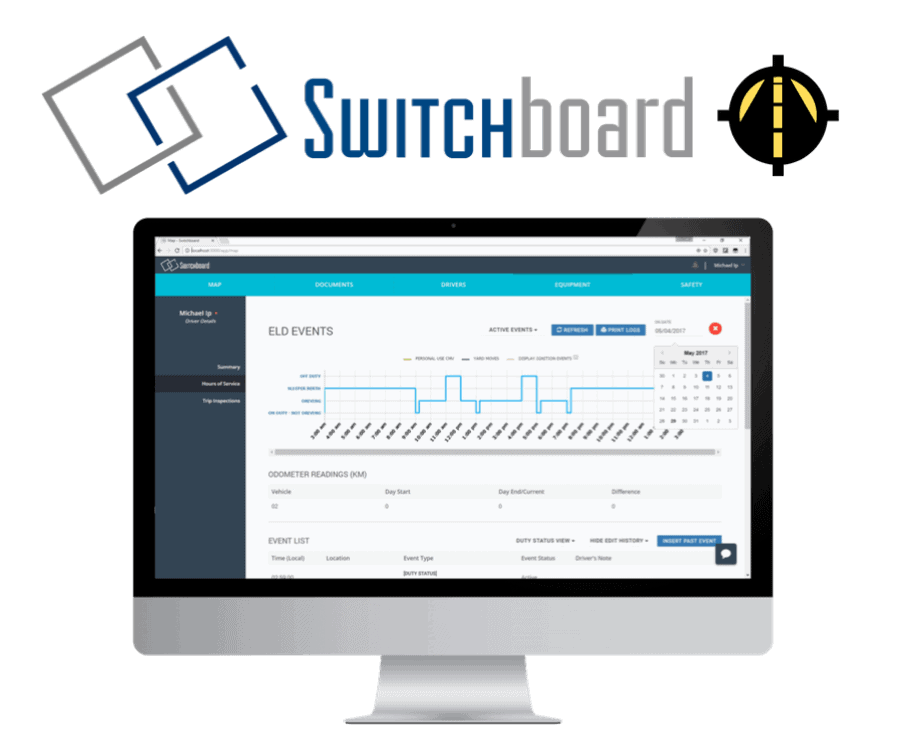The image depicts a computer monitor with a silver stand, showcasing the interface of a website called Switchboard. At the top of the monitor, there's the logo consisting of two intertwined squares, one gray and the other blue, slanting upwards to the right. The word "Switchboard" is displayed prominently, with "Switch" in blue and "Board" in gray. Next to it, there is a distinct circular logo featuring black protrusions and a yellow graphic. The website interface displayed on the monitor appears white, gray, and blue, with various graphs, lines, numbers, and dates. On the right side, there is a section titled "ELD events" along with a check icon at the bottom right.

Overall, the image is set against a white background, featuring detailed elements of a typical computer display, possibly in a work, home, or school setting.